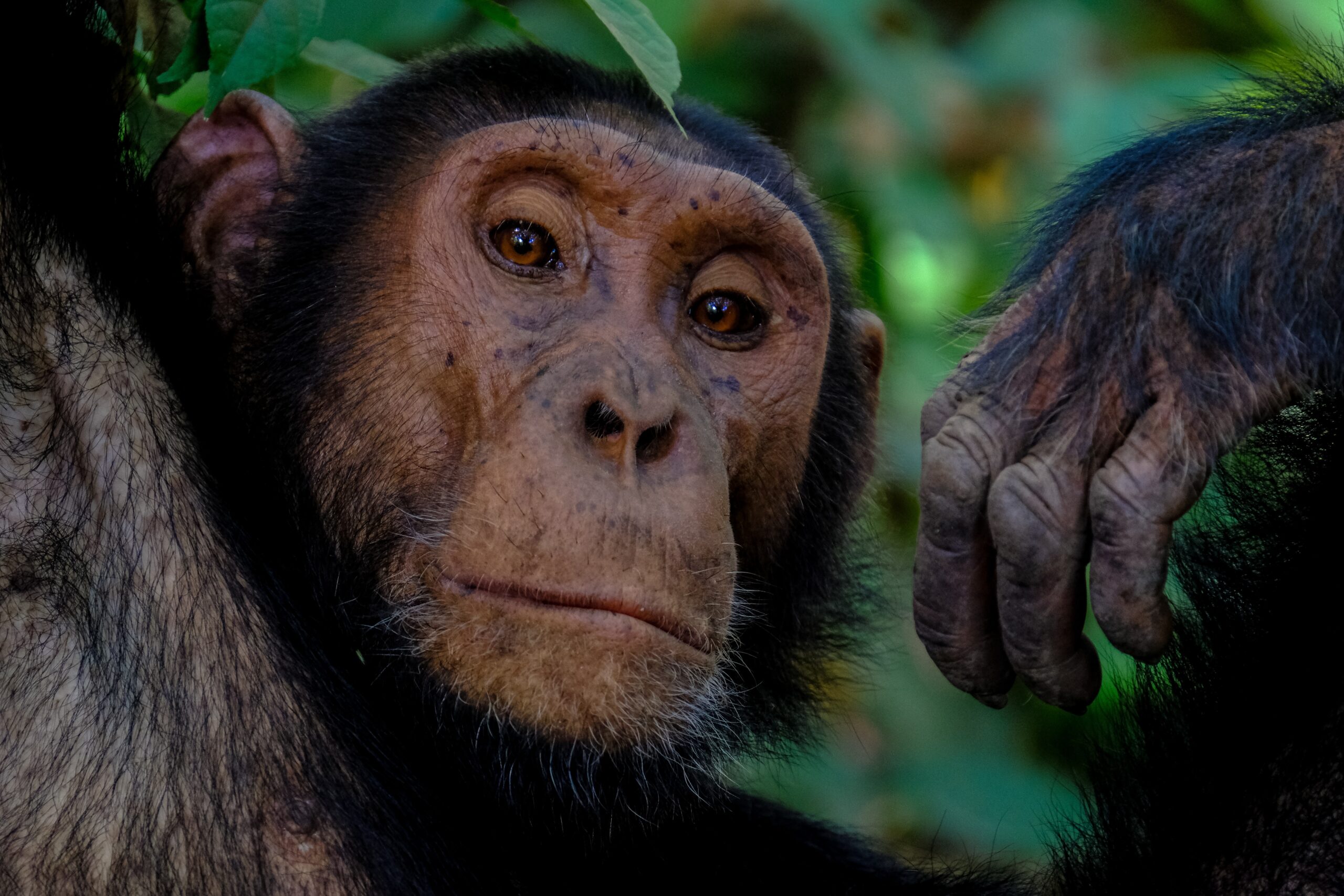This landscape, high-resolution portrait captures the face of a chimpanzee in meticulous detail. The chimpanzee, notable for his serious and contemplative gaze, directs his deep brown eyes—encircled by black pupils—straight into the camera. His head, shoulder, and left hand are prominently featured, with his hand resting relaxed by his face. Sparse hair dots his face, with more pronounced black and graying fur surrounding it, forming what can be described as a graying beard. His nose and much of his face display distinct fur patches that highlight his expressive features.

The green, blurred backdrop, speckled with occasional yellow lights, hints at a jungle setting, with one solitary leaf adorning his forehead. His ears, especially the large one on the right, are prominently visible. Attention to his left arm reveals hair covering all the way down to his knuckle, where his fingers then appear hairless, wrinkled, and speckled. The chimpanzee’s apparent habitat and the meticulous level of detail underscore the professionalism of the photograph, capturing the subject's textured skin, inset eyes, and overall demeanor in striking clarity.